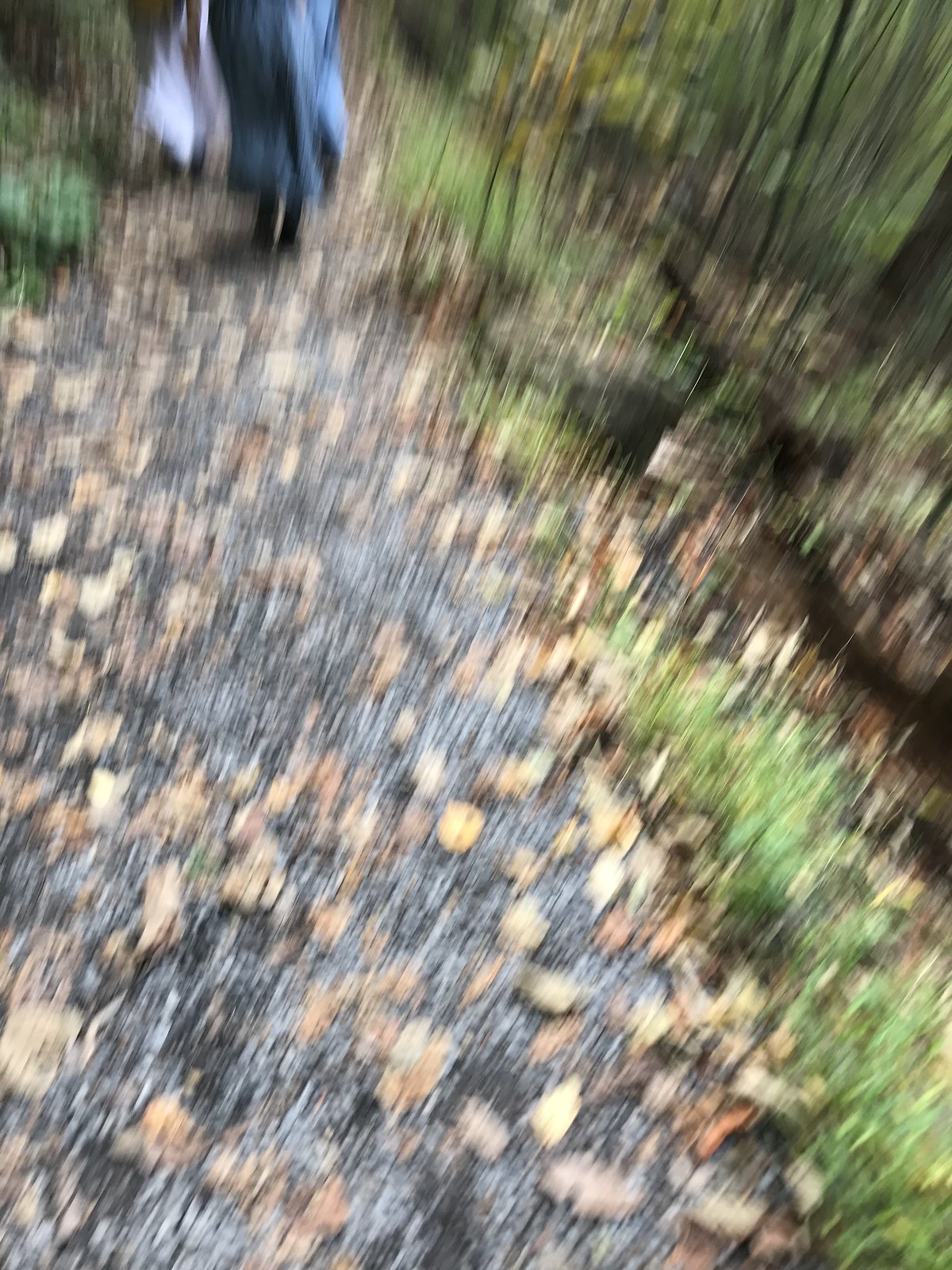This blurry photograph captures a serene, forested pathway covered with a mix of yellow, brown, and orange fallen leaves, hinting at an autumn scene. The road, made of concrete stone, appears somewhat wet, adding to the sense of a recent rain or dampness. Although unfocused, one can faintly discern a person in blue attire, perhaps a jean skirt, with dark pants. This person, holding an indistinguishable object on their left shoulder, walks along the pathway positioned more to the left side of the image. Surrounding this path are scattered patches of green vegetation and taller bushes, albeit unclear due to the blurriness. To the top right side of the photograph, there's a noticeable raised surface, possibly a rock, and hints at a body of water, like a small river or lake.